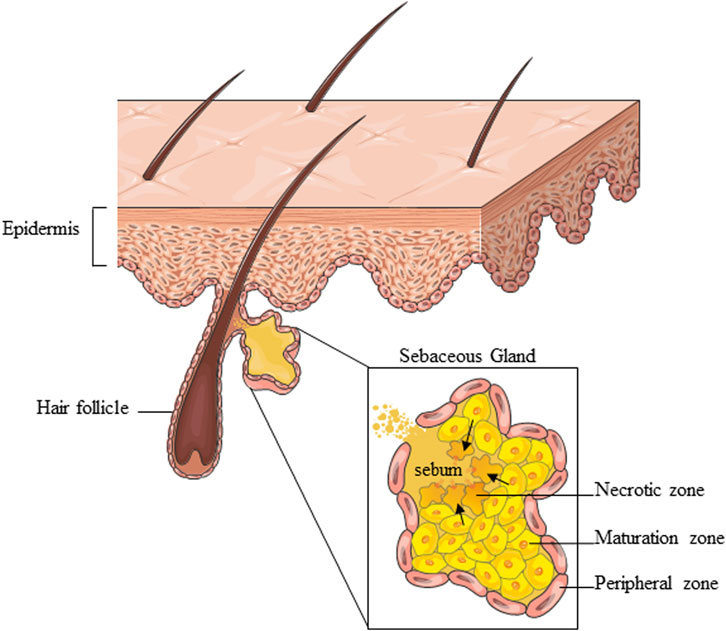In this detailed scientific illustration from a textbook, we observe a cross-section of human skin, prominently labeled at the top as the "epidermis." The light pink epidermis layer is depicted with undulating contours, suggesting the dynamic nature of skin cells. Protruding from the epidermis are four brown hair follicles, each extending beneath the skin surface. One hair follicle is particularly detailed, showcasing its structure and being specifically labeled.

Located beneath the epidermis, a rectangular magnified area highlights a sebaceous gland. This gland is composed of various zones: the necrotic zone, the maturation zone, and the peripheral zone, with each zone distinctly colored and labeled. The gland itself is primarily yellow, with cells in the maturation and peripheral zones depicted in shades of pink and yellow. At the core of the gland, "sebum" is indicated, highlighting its role in producing and secreting this oily substance. The intricate network of zones within the sebaceous gland is outlined with thin black lines, emphasizing the complex cellular structure that underscores its function in maintaining skin and hair health.